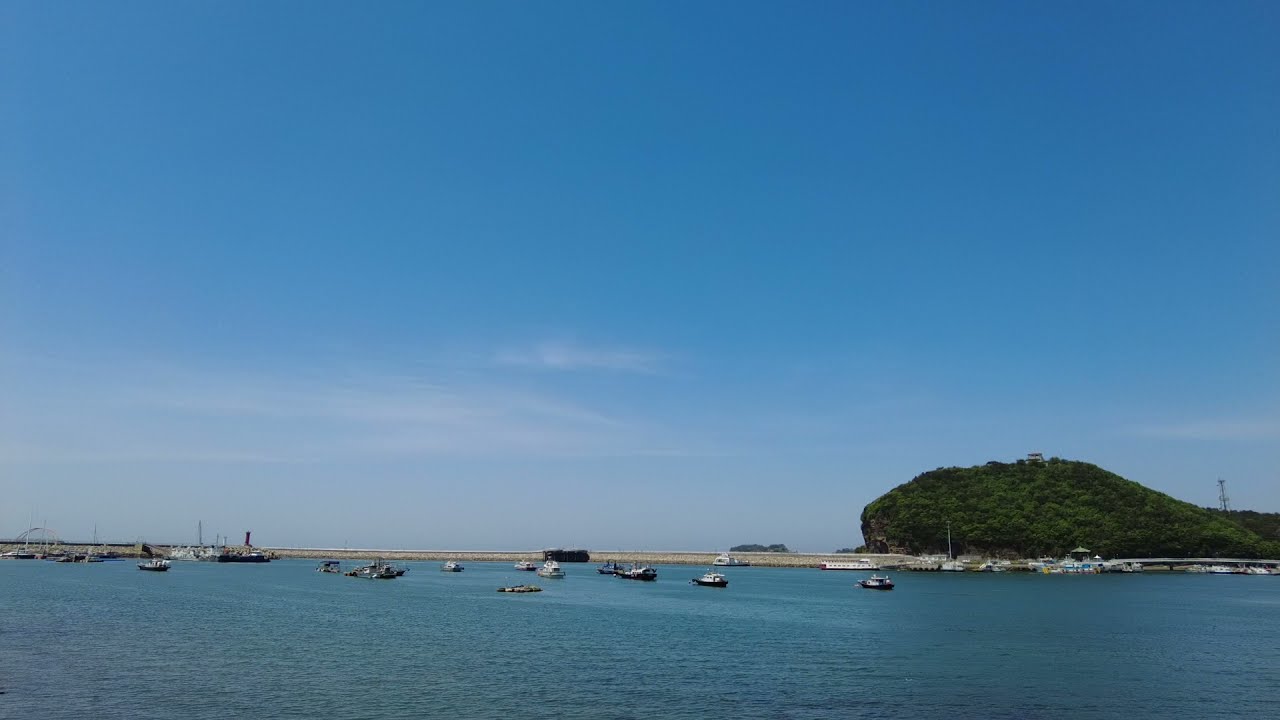This horizontal rectangular photograph showcases a scenic lake area taken from the shoreline. The foreground consists entirely of water, leading the eye to a collection of anchored boats in the distance. Most of these boats are white with black hulls. Farther out, a prominent seawall stretches across the image, featuring an opening underneath and culminating at a lighthouse. Behind this seawall, a bridge spans from the very left to the very right of the photograph.

On the right side of the image, a land structure rises approximately 50 feet above the bridge and boats. This hill is mostly covered in lush green vegetation, with only the lower rocky part visible. The top of the hill is densely packed with trees and bushes.

Dominating about 80 percent of the background, the sky transitions from a dark blue at the top to lighter shades near the horizon, where thin, wispy clouds are scattered.